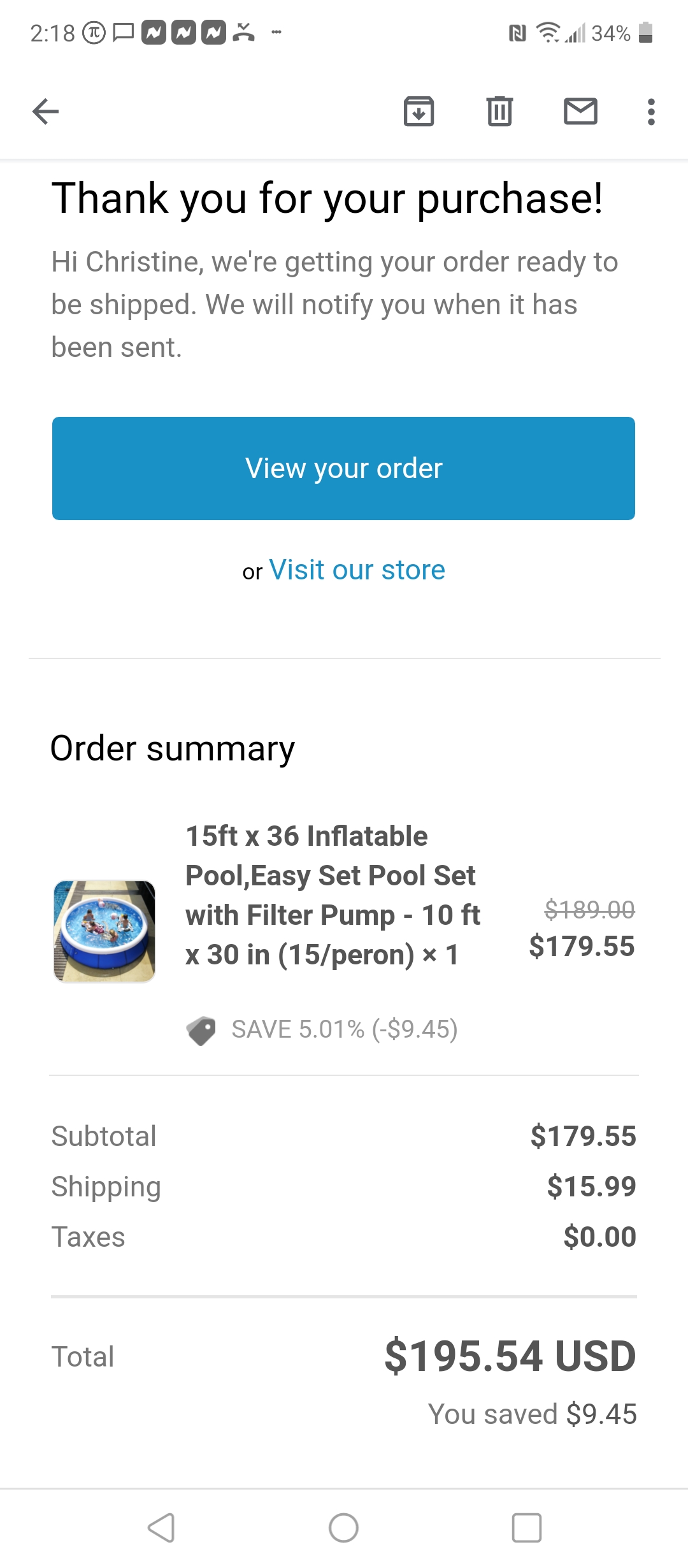Screenshot of an Order Summary from an Online Store:

The image is a screenshot of an order confirmation email received through Google Mail from an online store. The email begins with a thank you message: "Thank you for your purchase." Below this, the store addresses the customer, Christine, informing her that her order is being prepared for shipment and will be notified once it is sent.

The top section of the email includes a prominent blue "View Your Order" button and a "Visit Our Store" link. 

Following this, the order summary is displayed, detailing the items purchased. Christine has ordered a 15 by 36 feet inflatable pool, which comes equipped with a filter pump. The original listed price of the pool was $189, which is visibly crossed out. The discounted price is now $179.55, reflecting a savings of $9.45 (5.01%).

Below the item details, the cost breakdown is as follows:
- Subtotal: $179.55
- Shipping: $15.99
- Taxes: $0.00
The total amount for the purchase is $195.54 USD.

The background of the email is white, providing a clean and clear presentation of the information.